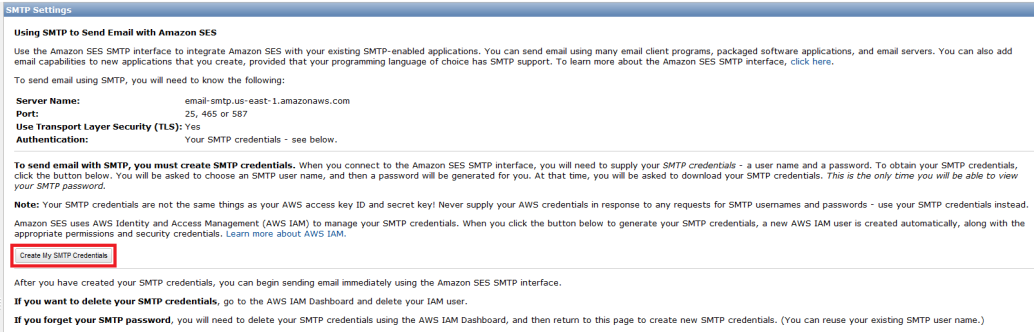The image provides detailed information regarding SMTP settings for using Amazon Simple Email Service (SES). The title "SMTP Settings" is prominently displayed within a blue border at the top. Below this, on a white background, the text outlines how to use the Amazon SES SMTP interface to send emails.

The instructions state that Amazon SES can be integrated with existing SMTP-enabled applications, allowing users to send emails using various email client programs, packaged software applications, and email servers. Additionally, new applications with SMTP support can also utilize this service.

To learn more about the Amazon SES SMTP interface, a clickable option is provided. The steps to send an email using SMTP are then detailed:

1. **Server Name:** `email-smtp.us-east-1.amazonaws.com`
2. **Port Numbers:** 25, 465, or 587
3. **Use Transport Layer Security:** Yes
4. **Authentication:** Your SMTP credentials (details provided below)

The text emphasizes that users must create SMTP credentials to connect to the Amazon SES SMTP interface. These credentials include a username and password. To obtain them, users are directed to click a button labeled "Create My SMTP Credentials," which is highlighted with a red block. Upon doing so, users will be guided to select an SMTP username and generate their credentials. A critical note mentions that this is the only time users will be able to view their SMTP password, thus highlighting the importance of downloading the credentials immediately.

This caption accurately conveys the essential details provided in the image regarding SMTP settings for utilizing Amazon SES.